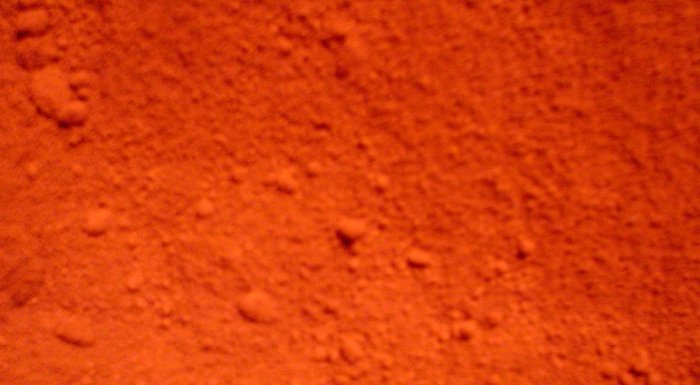This close-up image features a textured, rust-colored surface that could either be a granular material like powder or a rugged natural object, such as dirt or rock. The image's surface is mostly consistent in its earthy, reddish-brown color with elements that suggest a powdery substance. The overall texture appears uneven, with clusters of small, rounded chunks scattered throughout. These clusters are especially prominent in the upper left-hand corner and the center of the image, where larger fragments and clumps are concentrated. In contrast, the upper right-hand corner is noticeably smoother and less textured, appearing almost blurry with finer particles. The fine-grained powder here extends across the entire upper right section, setting it apart from the slightly coarser granules and pebble-like formations elsewhere. The material could be interpreted as a rusted surface, powdered dirt, or even an image of the Martian landscape, given its deep orange to red hue and the varied texture that includes divots and holes throughout.